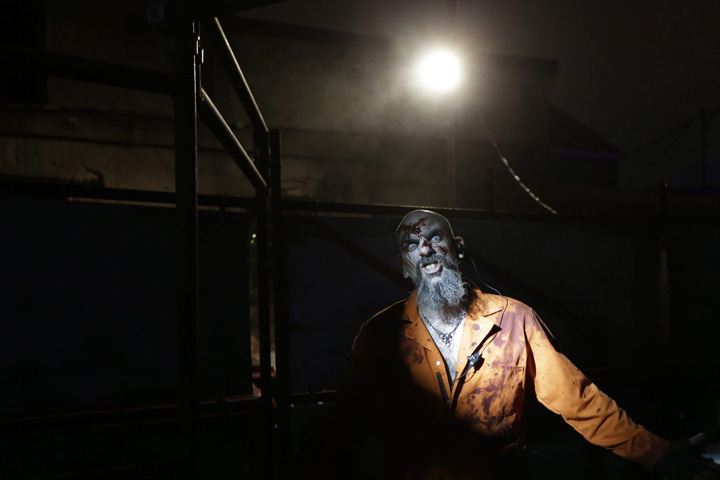The image is a dark, atmospheric scene that evokes a sense of horror, set in what appears to be a derelict warehouse. The setting is dominated by shadows, with only a sliver of light illuminating a menacing figure at its center. This man has a barren scalp, piercing blue eyes, a gray beard, and a mustache, all smeared with either dirt or blood, adding to his formidable appearance. He wears a yellow-orange jacket or jumpsuit, only partially buttoned, revealing a bare chest underneath. The garment is splattered with what looks like blood, contributing to the overall grim atmosphere. An eerie light source situated above him casts an unsettling glow, highlighting his menacing expression. Next to him is a metal structure composed of vertical and horizontal poles, adding to the industrial decay of the scene. The image strongly evokes the atmosphere of a horror movie, instilling a sense of dread and tension.